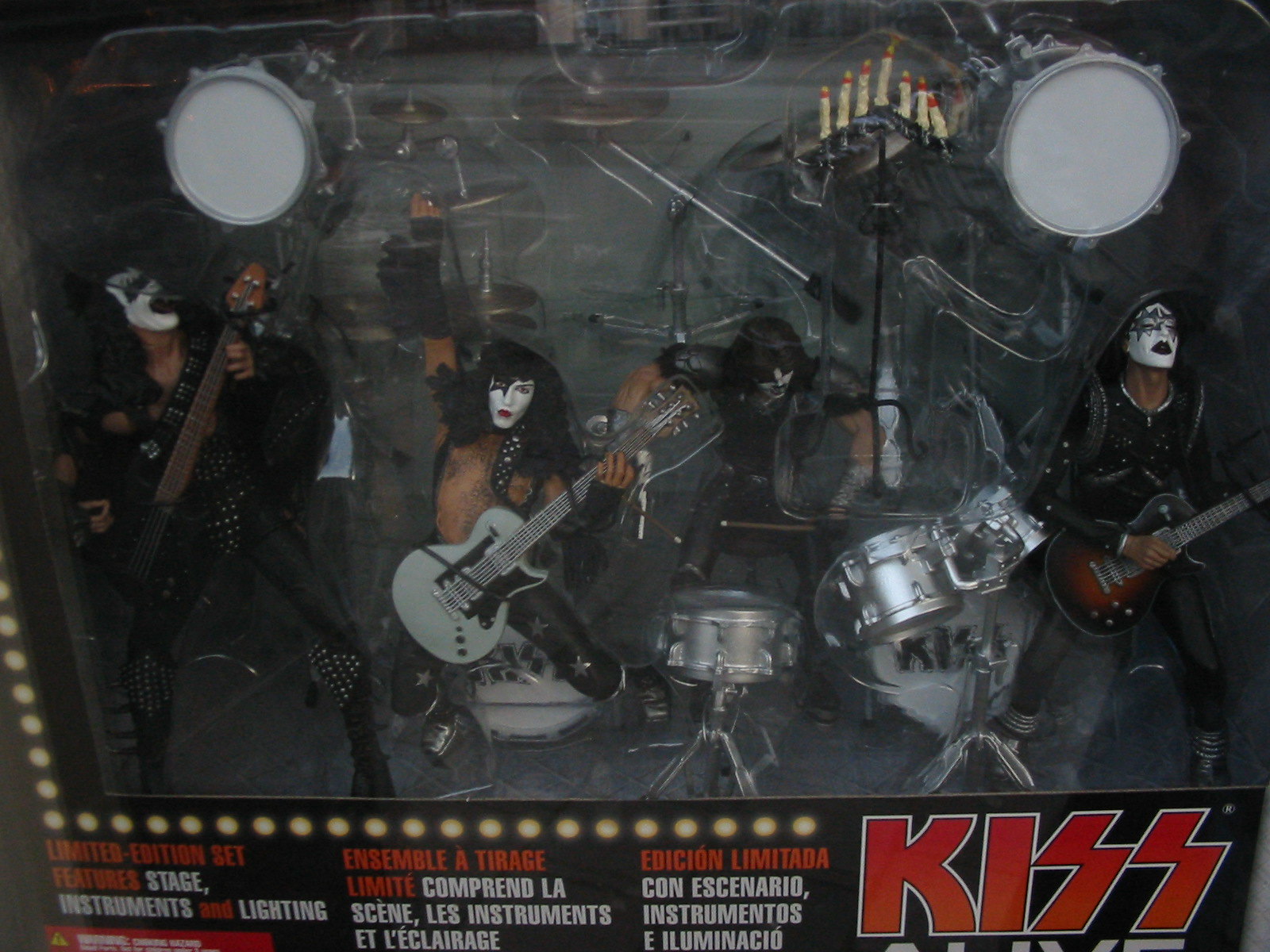In this rectangular image, we see a detailed photograph of a box containing action figures of the legendary rock band KISS. Each band member is meticulously sculpted and painted, capturing their iconic white and black kabuki makeup with red lips and black eyeliner. The figures are posed in full performance mode, with Gene Simmons prominently featured on the left, famous for his tongue sticking out, a guitarist mid-jump in the middle, the drummer behind a silver drum set, and another guitarist on the far right. They are equipped with their respective instruments and additional stage props, including a set of candles and yellow stage lights lining the bottom and sides. The see-through packaging showcases the figures in transparent plastic, along with text below them that reads "Limited edition set, features stage, instruments, and lighting," also translated into multiple languages including Spanish and French. The word "KISS" is emblazoned in bold red block print in the lower right corner. This carefully detailed collectible set is a homage to the band's electrifying stage presence.